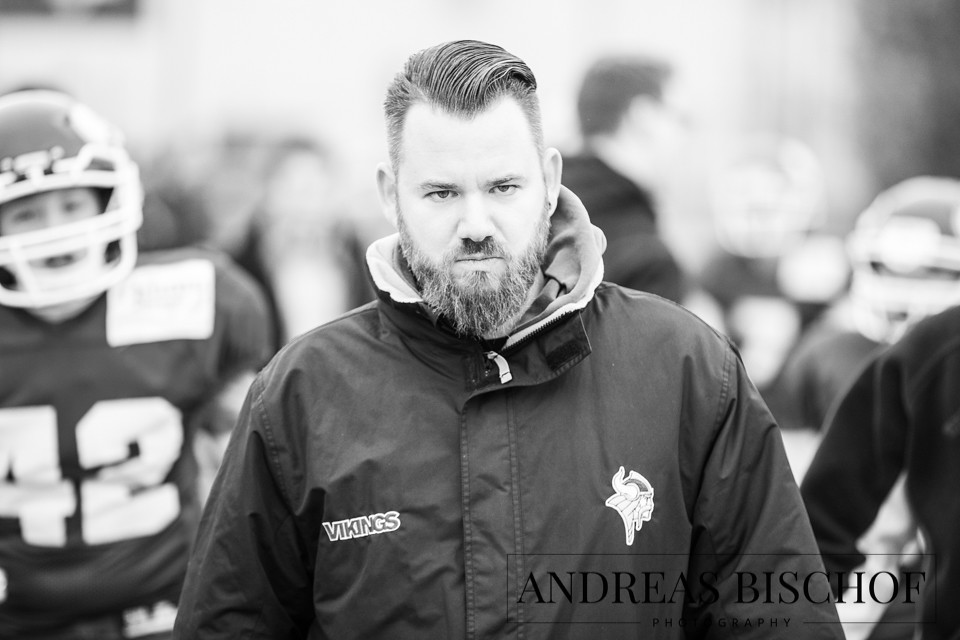A high-quality black-and-white photograph features a central figure who appears to be a young Caucasian man with medium-length hair and a beard, displaying a serious expression. He wears a dark hoodie-style jacket with the "Vikings" logo on the left chest and the team name written on the right. In the background, blurred football players in their uniforms and helmets are visible, adding to the sports context of the image. Some additional non-uniformed individuals are also present, blending into the bright yet indistinct backdrop. At the bottom right corner of the photograph, the name "Andreas Bischoff" is clearly written in black capital letters, identifying the photographer.